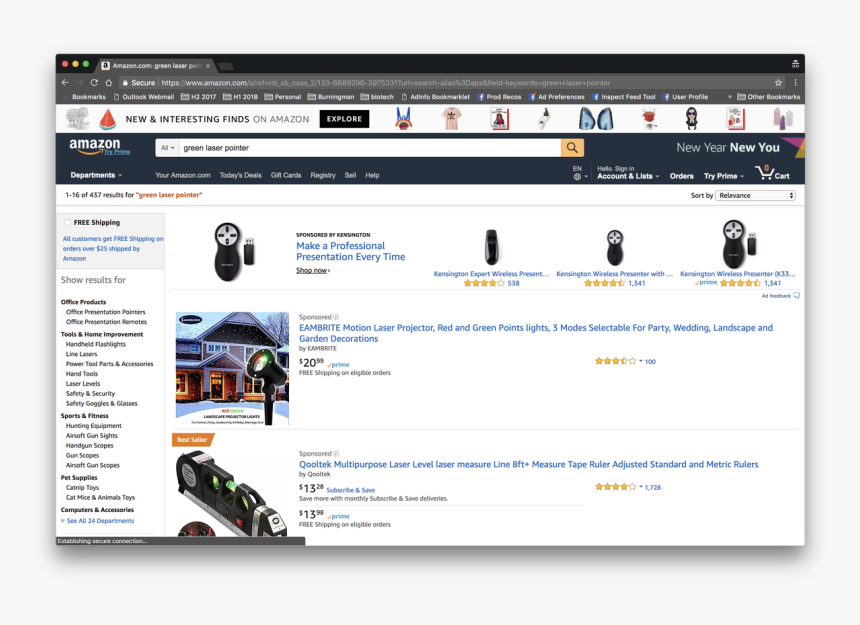**Caption:**

The webpage on display is Amazon.com, a secure website marked by the lock icon beside the URL. At the top, the iconic Amazon logo is visible. The page highlights "New and Interesting Finds on Amazon" with a prominent black "Explore" button underneath. Following this section, the Amazon logo appears again alongside "Prime."

Beneath the logos, there's a search bar with the text "green laser pointer" already entered. To the right of the search bar, a notable banner reads "New Year, New You." Below, the page reveals the search results, displaying "1-16 of 436 results for 'green laser pointer'."

The results section features several items including the following:

1. **Sponsored: Kingston Expert Wireless Presenter**
   - **Rating:** 4 out of 5 stars from 538 reviews.
   - **Details:** Kingstons Wireless Presenter with a rating of 4.5 out of 5 stars from 1,341 reviews.
   - **Prime Eligibility:** Yes.

2. **Sponsored: Embrite Motion Laser Projector**
   - **Description:** Red and green points of light with three selectable modes for party, wedding, landscape, and garden decoration.
   - **Price:** $20.99.
   - **Prime Eligibility:** Free shipping on eligible orders.
   - **Popularity:** Bestseller.

The page also notes that free shipping is available for all customers on orders over $25 when shipped by Amazon. The visual presentation of the suggested products emphasizes professional quality and user convenience, showcasing Amazon's extensive catalog and services.